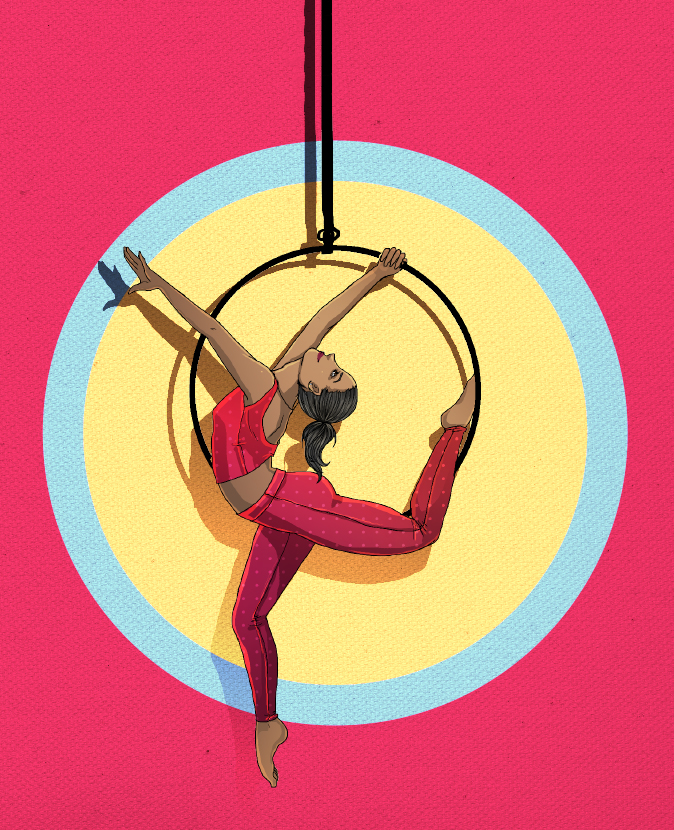The artwork depicts a young acrobat contorted into a bow-like, arabesque position within a metal hoop suspended by a rope, presumably from the ceiling. She is clad in a red leotard and is barefoot, with her head bent backwards. Her left arm extends upwards at a 45-degree angle, while her right arm is stretched straight along her torso to grasp the hoop. Her left leg bends backwards towards her head, with her left foot bracing against the inside of the hoop, as her right leg hangs straight down, aligned with her body. The background features a bullseye pattern with an outer ribbed layer of magenta, followed by a sky-blue ring, and a pastel yellow dot in the center, drawing focus to the acrobat's centered position in the artwork. This image, a detailed drawing, captures the grace and flexibility of the acrobat in a dynamic aerial pose.